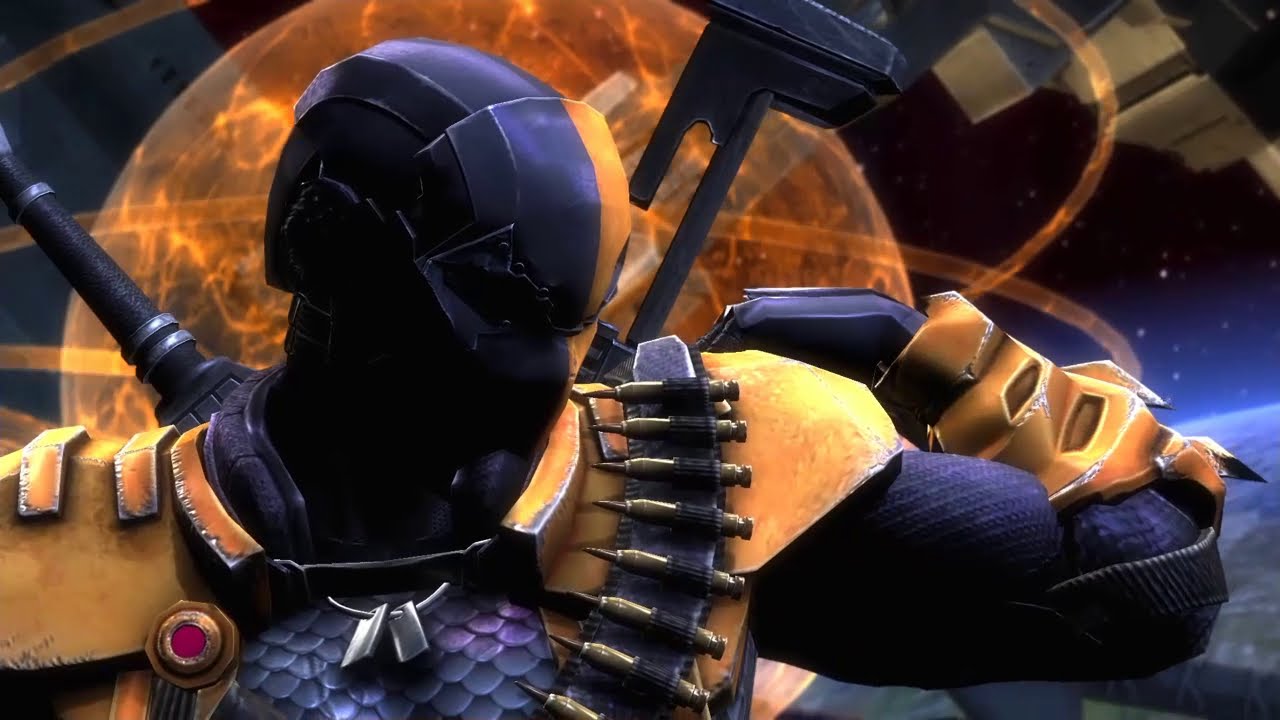A highly detailed digital image of a video game or animated movie character, showcasing a man clad in intricate armor. His face is obscured by a full-coverage mask made of dark black metallic material with subtle blue hues at the top, creating a shadowed effect on the sides of his face and neck. His shoulder armor is predominantly orange, accented with hints of yellow, and underlines his formidable presence. A string of bullets, held in a bandolier, cascades from his right shoulder across his chest, adding to his battle-ready appearance. He wears light silver dog tags around his neck.

The character's attire includes a dark blue and purple scaled shirt underneath the armor, with his visible right arm adorned in dark material with purple tones and lines sloping upwards. On his right shoulder and arm, he also sports orange guards, further enhancing his rugged look. Various weapons are seen behind him, suggesting his readiness for combat.

In the background, a large, fiery sphere reminiscent of a sun or a giant orange planet dominates the scene, surrounded by spiral lines that give it an atomic structure appearance. The background transitions into a dark blue and indigo expanse, dotted with tiny star-like lights, creating the impression of a space setting with a nearby planet just visible to the right and center, bathed in cosmic light.